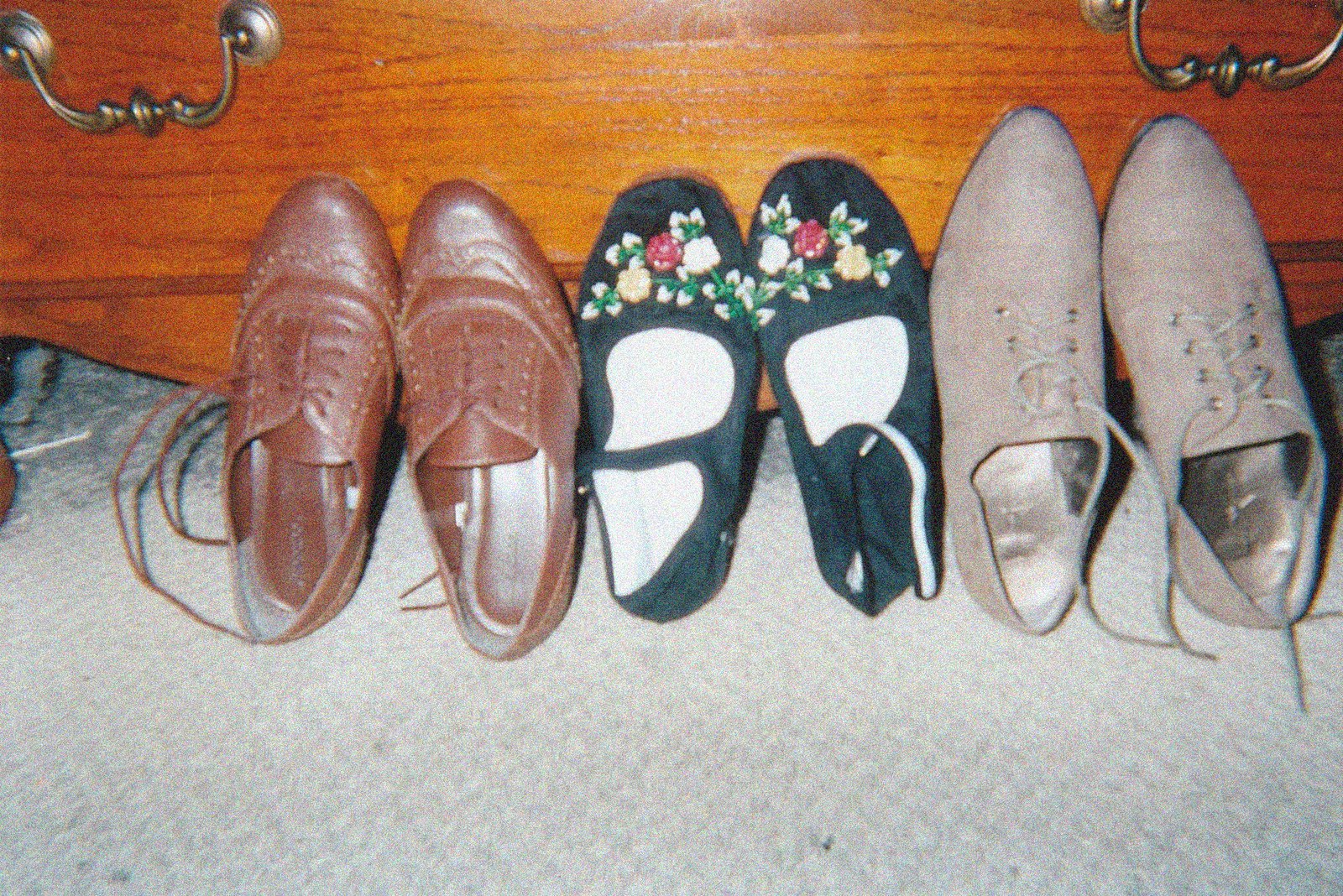This photograph captures three distinct pairs of shoes leaning on their heels against a reddish-brown dresser with brass handles, set on a grey diamond-patterned carpet. On the left, a pair of brown leather dress shoes with thin laces and imprints along the sides; in the middle, ornate black slip-on shoes adorned with a delicate floral embroidery featuring red, yellow, and white flowers amid green and white-tipped leaves, connected by a black band at the ankle; and on the right, a pair of sandy-colored, suede-like dress shoes with laces and a satin interior, all reflecting a somewhat vintage style.